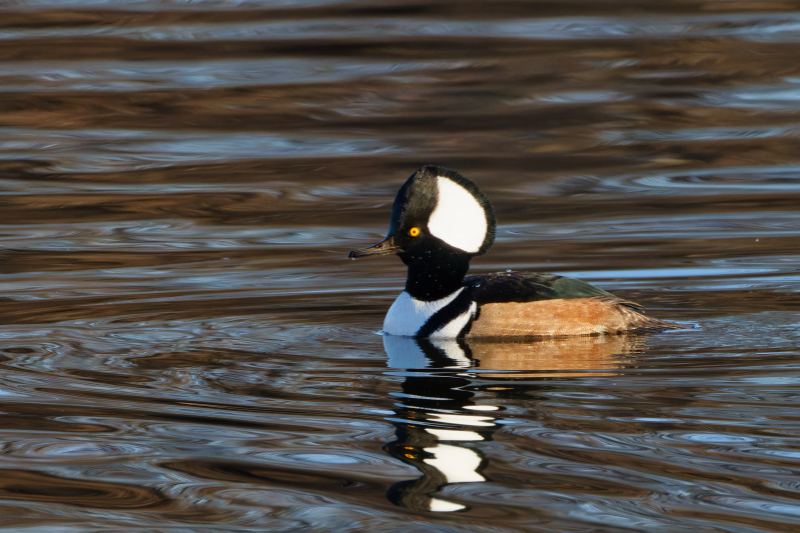The close-up photograph captures a duck swimming in brown, ripply water on a sunny day. The duck is positioned sideways in the center of the image, facing to the left, with its eye visibly orange or yellow. The duck's head is primarily black with a prominent white spot at the back, while a black stripe runs down its neck. It has a brownish-dark beak and a chest that's both white and marked with a black stripe. The body is black, transitioning to lighter brown on the sides and possibly accented with a hint of green. Notably, the water reflects the duck’s head, neck, and chest. Only the duck and its reflection are captured against the wavy, sunlit water, with no shore or sky visible in the composition.